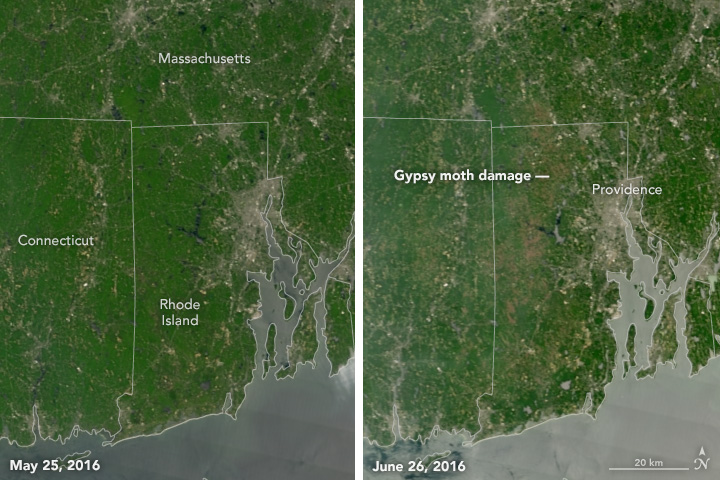The image is a rectangular aerial or satellite view comparing gypsy moth damage over New England. It is divided into two almost square sections with a vertical white line about half a centimeter thick. The left image, dated May 25, 2016, shows the states of Massachusetts, Connecticut, and Rhode Island in vibrant green with clearly indicated state lines and fine details like rock formations, water bodies, and coastlines. The right image, dated June 26, 2016, displays the same area with noticeable brown patches indicating gypsy moth damage, particularly evident around Providence. Additional annotations include a label "Gypsy Moth Damage" on the vertical white line, a 20-kilometer scale bar, and a north arrow for orientation. Both maps are detailed, using white text and various distinctions to aid in the visual comparison of the landscape over a month's interval.